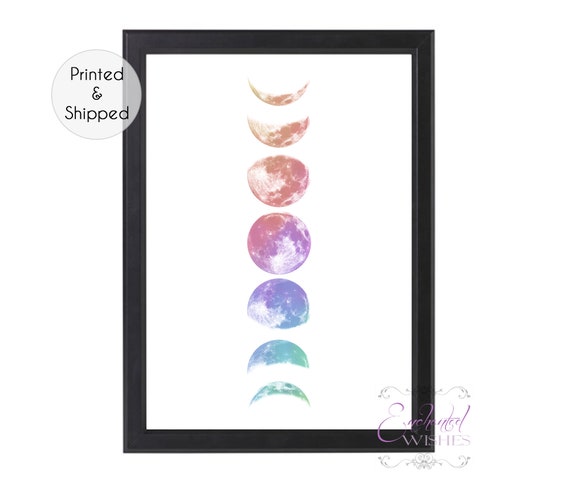This is a photograph of an artistic watercolor painting framed in black. The central focus of the image depicts various phases of the moon arranged in a vertical sequence on a white background. Starting at the top, the moon appears as a slender crescent in yellow-orange hues. As the phases progress downward, the colors transition smoothly through an ombre effect, from red and purple at the top to a full moon in a mix of orange, pink, and purple in the middle. Below the full moon, the colors continue to blend into cooler tones of green, blue, and finally a greenish-blue for the bottom crescent moon. Each lunar phase is depicted in a blend of colors that gradient from one to the next, reminiscent of the colors of the rainbow.

The black frame is about an inch thick, providing a stark contrast to the white backdrop. Additionally, toward the top left corner, there is a light gray, slightly transparent circle outlined in black that reads "printed and shipped." In the bottom right corner, there is a cursive, possibly embroidered label that says "enchanted wishes" in pink and gray text with a swirly, decorative design. The overall composition of the framed painting evokes the enchanting progressions of the moon, blending art and cosmic beauty seamlessly.